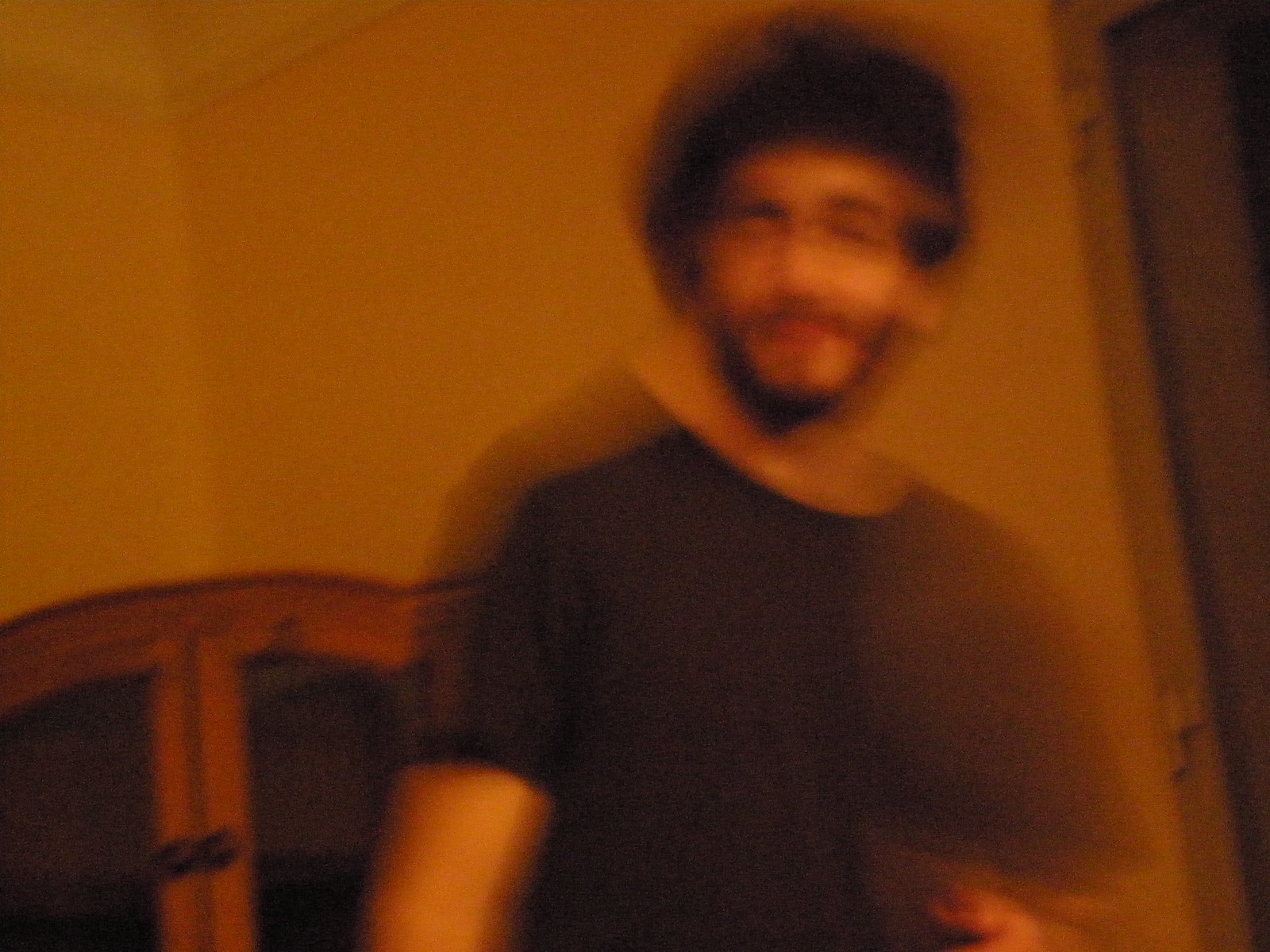This image is a blurry photograph taken inside a house, featuring a man standing near the corner of a wall. The man has fluffy, black afro-like hair, dark black eyebrows, and a short beard. He is wearing a black short-sleeved t-shirt and is looking slightly to the left. His eyes appear almost closed due to the blurriness of the image. The wall behind him appears beige but may reflect an orange hue from the lighting. To the bottom left of the image, there's an arch-shaped cabinet with two doors and round wooden knobs. To the right of the man, there's an open doorway.